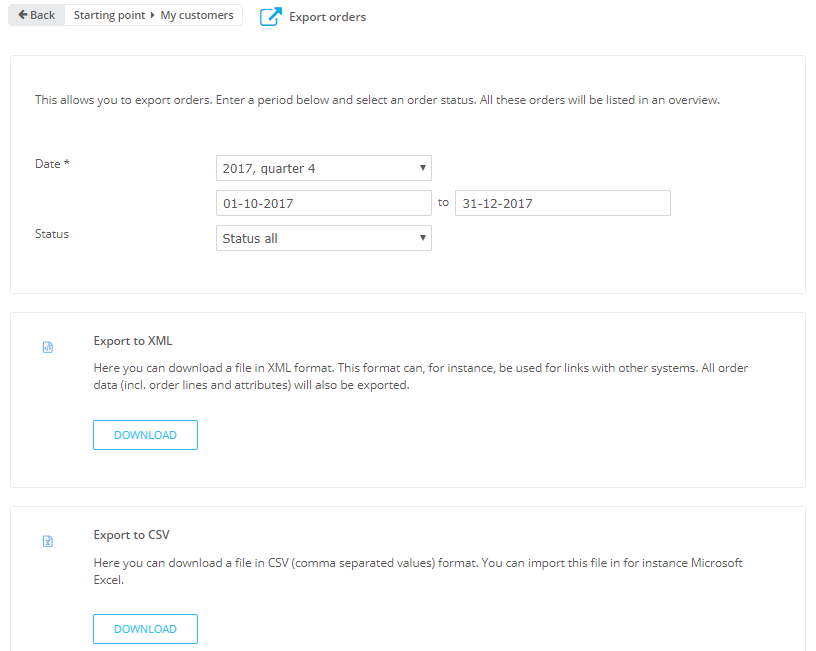The screenshot of the computer interface features a detailed and structured layout for exporting customer orders. At the top of the screen, a back button is positioned on the left, followed by a play button symbolized by a right-pointing triangle. Next to these controls, the screen title "My Customers" is prominently displayed. To the right, there is a logo featuring an upward-right arrow enclosed in a square, accompanied by the text "Export Orders."

Beneath this header, a rectangular information box provides instructions, stating, "This allows you to export orders. Enter a period below and select an order status. All these orders will be listed in an overview." 

The interface includes a date selection option on the left side, marked with an asterisk, suggesting that it is a required field. Users can input the date range using two adjacent input boxes labeled "From" and "To." 

Further down, a status dropdown menu labeled "Status All" is available, featuring a downward-pointing triangle to indicate additional category options.

At the bottom of the interface, two large rectangular sections are dedicated to export functions. The first section contains the "Export to XML" function, with a corresponding Download button. Directly below, the second section includes the "Export to CSV" function, along with its own Download button and a brief description of the export format. 

The organized layout is designed to guide users through the process of exporting customer orders efficiently, providing clear instructions and options at each step.